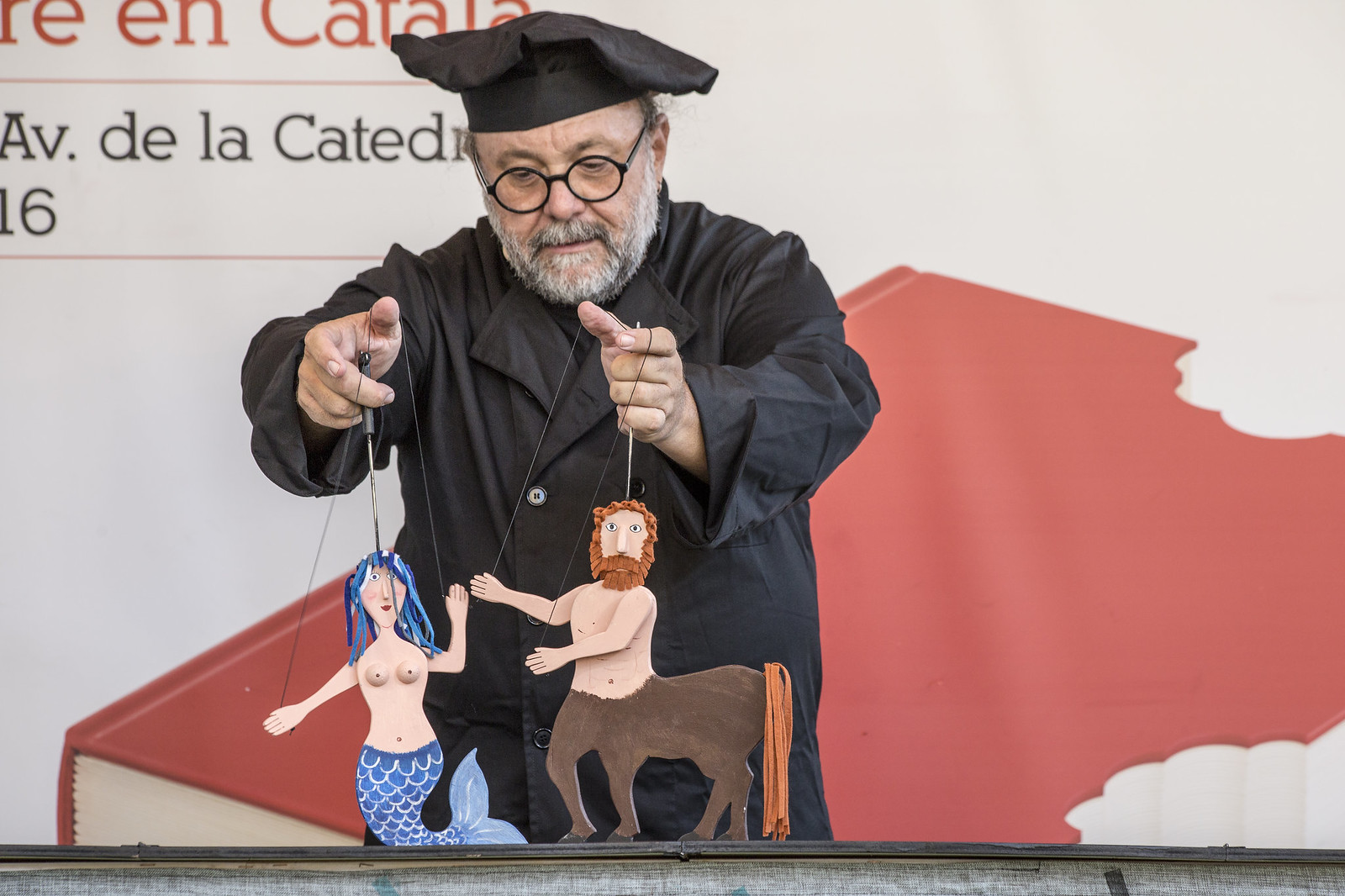In this color photograph, an older man with circular black frame glasses, a gray beard, a black chef-like outfit, and a matching hat stands at the center. He is positioned slightly to the left in a landscape-oriented frame, facing towards the camera with his arms extended, each hand manipulating a puppet. The man, evoking a professorial look, operates a topless wooden mermaid puppet with blue hair and a blue tail with his right hand. In his left hand, he controls a minotaur figure with an orange mane and human torso, also topless. Both puppets are suspended by strings, showcasing the man’s detailed control over their movements. Behind the man is a backdrop featuring a red book with bite marks on its sides, adding a whimsical element. The backdrop also includes text in the upper left corner, partially obscured and blurred, making it unreadable. The colors in the photo are vivid, including reds, off-whites, blues, browns, oranges, tans, and silvers, all contributing to the rich visual detail of the indoor scene.